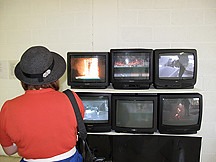The photograph appears to be an old image, possibly from the late 70s or early 80s, depicting a woman seen from the back. She is wearing a red short-sleeved shirt, a white belt, and blue bottoms. It's unclear whether she is wearing pants or a skirt as the image is cut off at the bottom. Her head is adorned with a gray, fedora-style sun hat with a black band and a pendant on it. She has neck-length brownish hair and a black shoulder purse slung over her right shoulder. The woman is intently watching six small television sets arranged on white shelves, three on the top shelf and three on the bottom. These TVs, likely considered high-tech at the time, display various channels, suggesting a section of a TV store against a backdrop of white painted concrete brick.